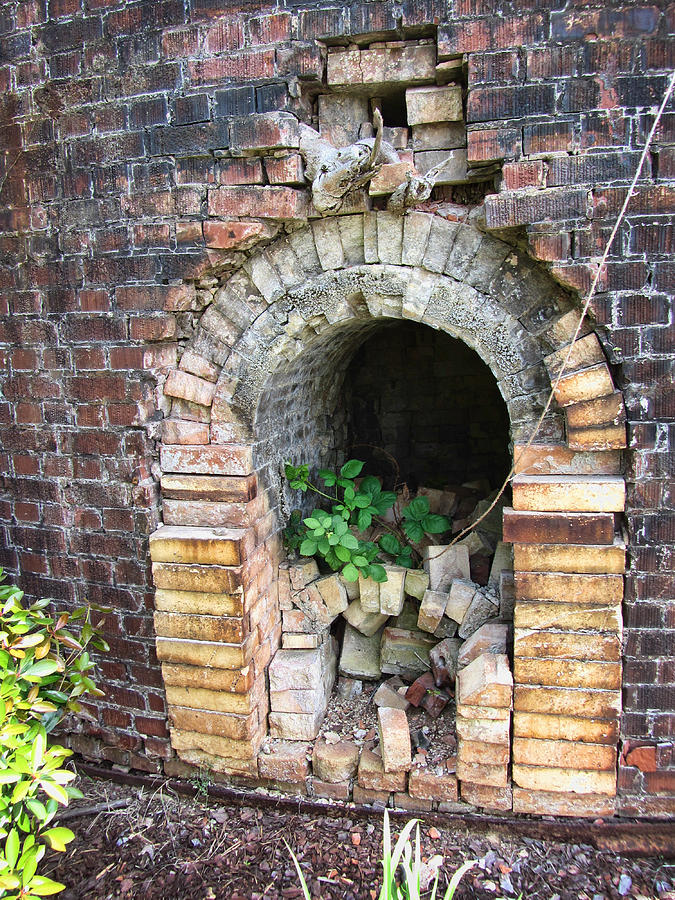In this realistic outdoor photograph oriented vertically, the setting features a dilapidated brick wall that appears either to be breaking down or under construction. The thick, dark red bricks, marked with blackened areas suggesting fire damage, form an intriguing backdrop. Centered within the wall is a small archway, possibly a vent, with an opening that leads into a tunnel. The archway, about 3 to 4 feet tall and 2 to 3 feet wide, is made of a different set of bricks; the arch's bricks are white and yellowed, forming a striking contrast against the main wall. Above the arch, the bricks are significantly decayed and collapsing, with some loose bricks and debris scattered inside the tunnel alongside a small bush.

In front of the wall, the ground is covered with wood chips or dead leaves, interspersed with green plants and high grass. A vine climbs the wall, adding to the scene’s decay and overgrowth. The overall atmosphere is one of forgotten history, as if this brick wall and its tunnel have withstood the test of time and elements, now overtaken by nature.